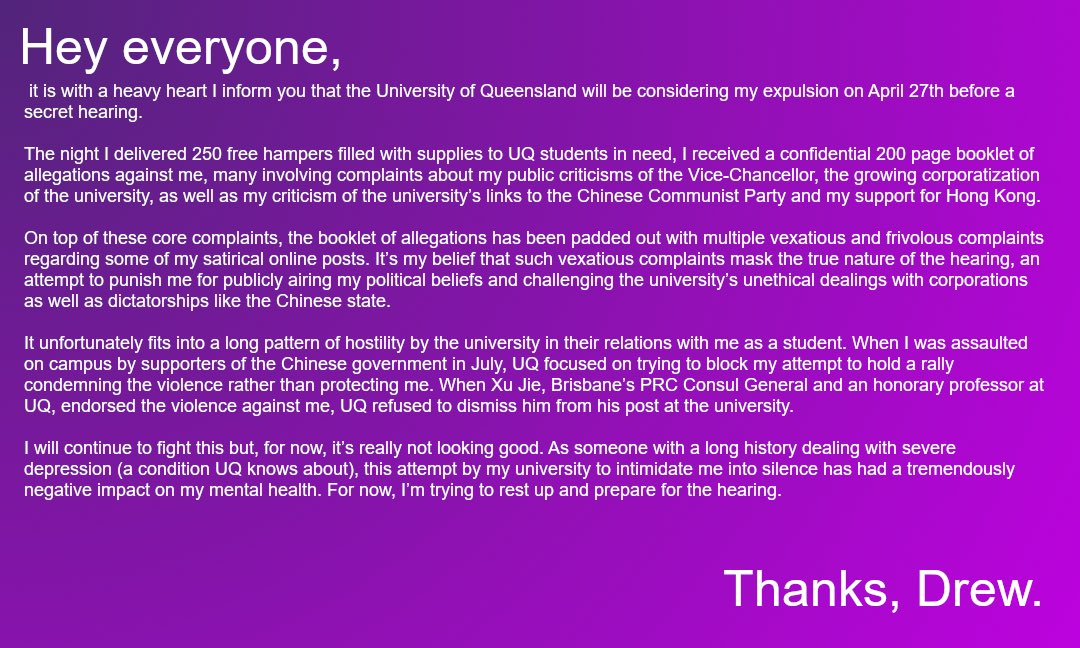This horizontally rectangular image serves as an announcement about a serious problem faced by an individual, Drew, involving potential expulsion from the University of Queensland. The background features a gradient of purple, darker on one side and lighter on the other, giving it a polished, almost presentation-like appearance. At the top, in bold white letters, it reads, "hey everyone." 

The main body of the message is composed of several paragraphs also in white text. The initial paragraph begins with, "It is with a heavy heart I inform you that the University of Queensland will be considering my expulsion on April 27 before a secret hearing." The narrative continues to describe a critical night when Drew delivered 250 free hampers filled with supplies to UQ students in need, only to receive a confidential 200-page booklet of allegations the same night. This booklet cites multiple complaints, many focused on Drew's public criticisms of the vice-chancellor, the increasing corporatization of the university, UQ's connections to the Chinese Communist Party, and Drew's support for Hong Kong.

Subsequent paragraphs elaborate on the contents of the allegation booklet, including not just core complaints but also a multitude of vexatious and frivolous ones concerning Drew's satirical online posts. Drew believes these complaints are attempts to mask the true intent of the hearing—to punish him for publicly voicing his beliefs and challenging the university's unethical dealings with corporations and dictatorships, such as the Chinese state.

The message also outlines a troubling history of hostility from the university. It mentions an incident in July when Drew was insulted by supporters of the Chinese government while attempting to hold a rally. Instead of focusing on protecting Drew or condemning the violence, the university seemingly prioritized halting his efforts. Additionally, when Zhu Zhibristain, the PRC consul general and an honorary professor at UQ, endorsed the violence against Drew, the university refused to remove him from his post.

Concluding this poignant message is a final paragraph, simply stating, "thanks, Drew," also in white text at the bottom of the image.